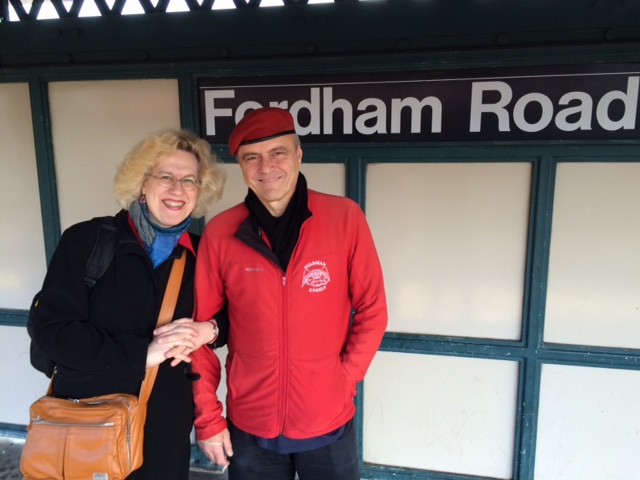In this detailed photograph, a man and a woman are standing in front of the Fordham Road subway station in New York City, against the recognizable backdrop of a white and green wall. The woman, who is blonde and wears glasses, is dressed for winter in a black coat with a blue scarf, and carries both a backpack and a large grey-brown overnight bag. Beside her is Curtis Sliwa, the founder of the Guardian Angels and a well-known radio talk show host. He stands out in his signature red beret and jacket, which features the Guardian Angels logo in white on the left chest. Under his jacket, he wears a blue shirt, paired with dark-colored pants. The familiar font of the Fordham Road sign and the background's dark green structures with white paneling firmly place this scene in a quintessential New York City subway station.